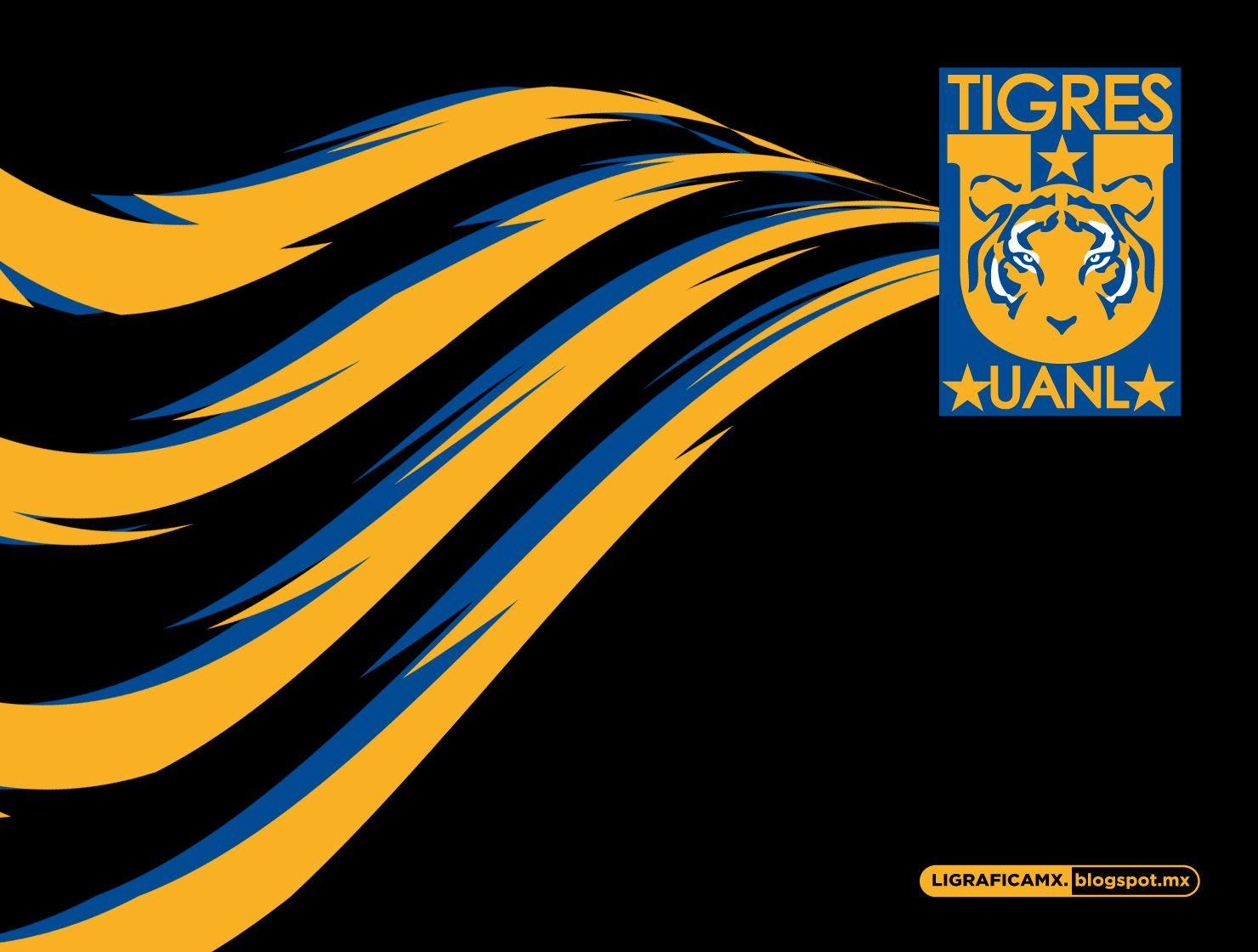This image features a modern and dynamic logo or banner, likely a poster or advertisement for a sports team. Dominating the scene is a striking logo situated in the upper right corner, set against a solid black background. The logo is rectangular and vertical, prominently displaying "TIGRES" in bold, capital letters at the top. Beneath this, a large "U", reminiscent of a collegiate font, is featured with a yellow star nestled between its legs. At the bottom of the "U" lies the illustration of a tiger’s face, rendered in dark blue and white.

Enhancing the dynamic nature of the design, jagged, wavy yellow and blue stripes sweep across the image from the bottom left to the top right, converging toward the tiger logo. These stripes are not straight but jagged, contributing to a sense of motion and energy, reminiscent of tiger stripes.

In the bottom section of the logo, the text "UANL" is flanked by stars on either side, all in capital letters. Towards the bottom right corner of the image, a yellow oval encloses the URL "LigaGraficaMX.blogspot.mx" in black type. The overall style is modern and illustrative, perfectly capturing the vibrant and energetic essence of the sports team it represents.